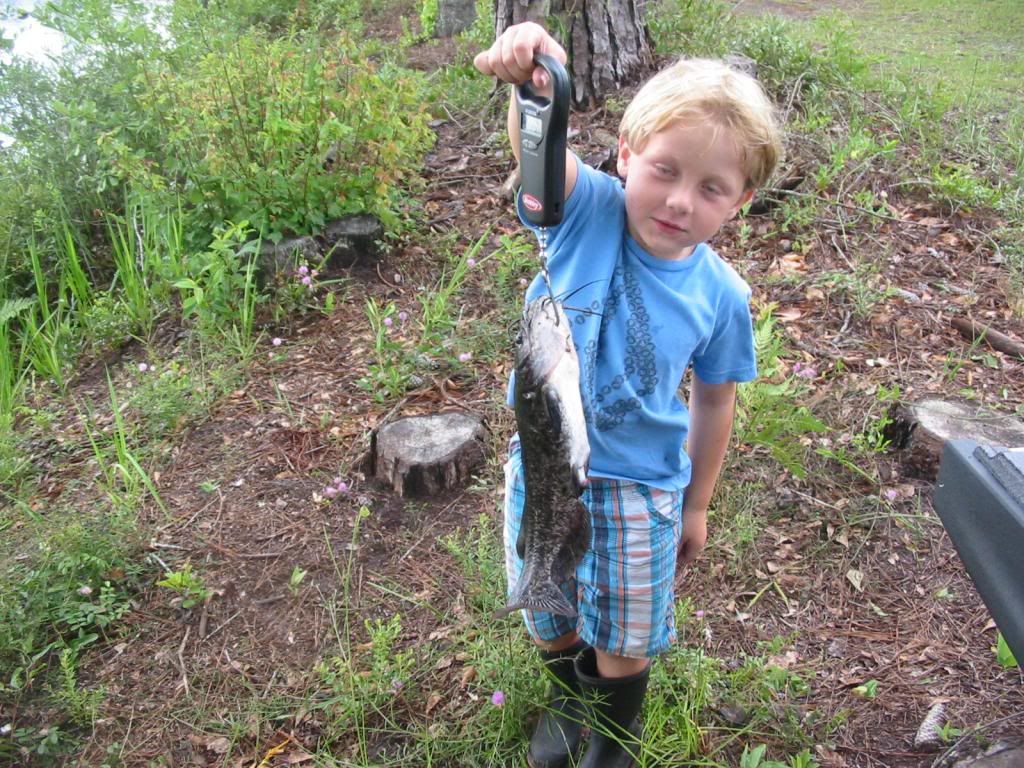In this photograph, captured in an outdoor setting, a small child with medium-length blonde hair stands at the center. The child’s eyes appear to be closed. He is dressed in a blue t-shirt that seems to feature a black design resembling seaweed. His outfit is completed with a pair of striped shorts in shades of blue and white and sturdy, black rubber boots that resemble waiter-style footwear, likely waterproof.

The child is holding a large catfish, which hangs by a plastic holder akin to a key fob or possibly a new type of fishing apparatus. The catfish, suspended on a sizable silver metal hook, displays a dark gray and white coloration, with distinct whiskers around its mouth.

The environment around the child suggests he might be in a yard, woods, or near a lake, though the exact location is ambiguous. A watermark indicating "Photobucket" spans over the image, accompanied by the phrase “protect more of your memories for less” in semi-transparent lettering, allowing a view of the image underneath but still readable.